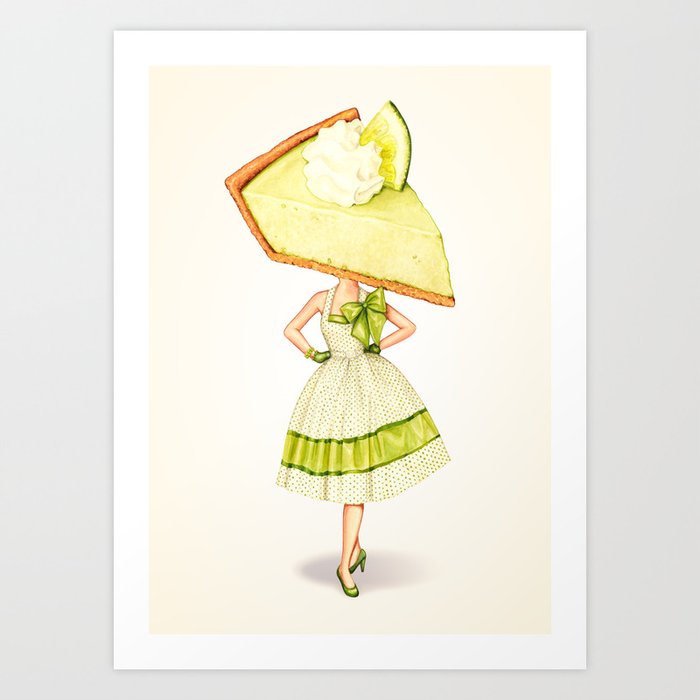This whimsical, cartoonish 1960s-style painting depicts a woman dressed in a striking, retro ensemble, with a unique twist—her head is replaced by an oversized slice of key lime pie. The key lime pie, featuring a biscuit base, a generous dollop of whipped cream, and a slice of lime on top, sits disproportionately larger than an actual head. The woman is adorned in a white, flared 1950s-style dress decorated with green polka dots and a prominent green ribbon running across the chest. Her outfit is further complemented by a horizontal green line near the hem, and she wears matching green high-heeled shoes and green gloves. The green elements of her attire—reminiscent of the vibrant key lime pie—create a harmonious color palette that ties the entire image together.